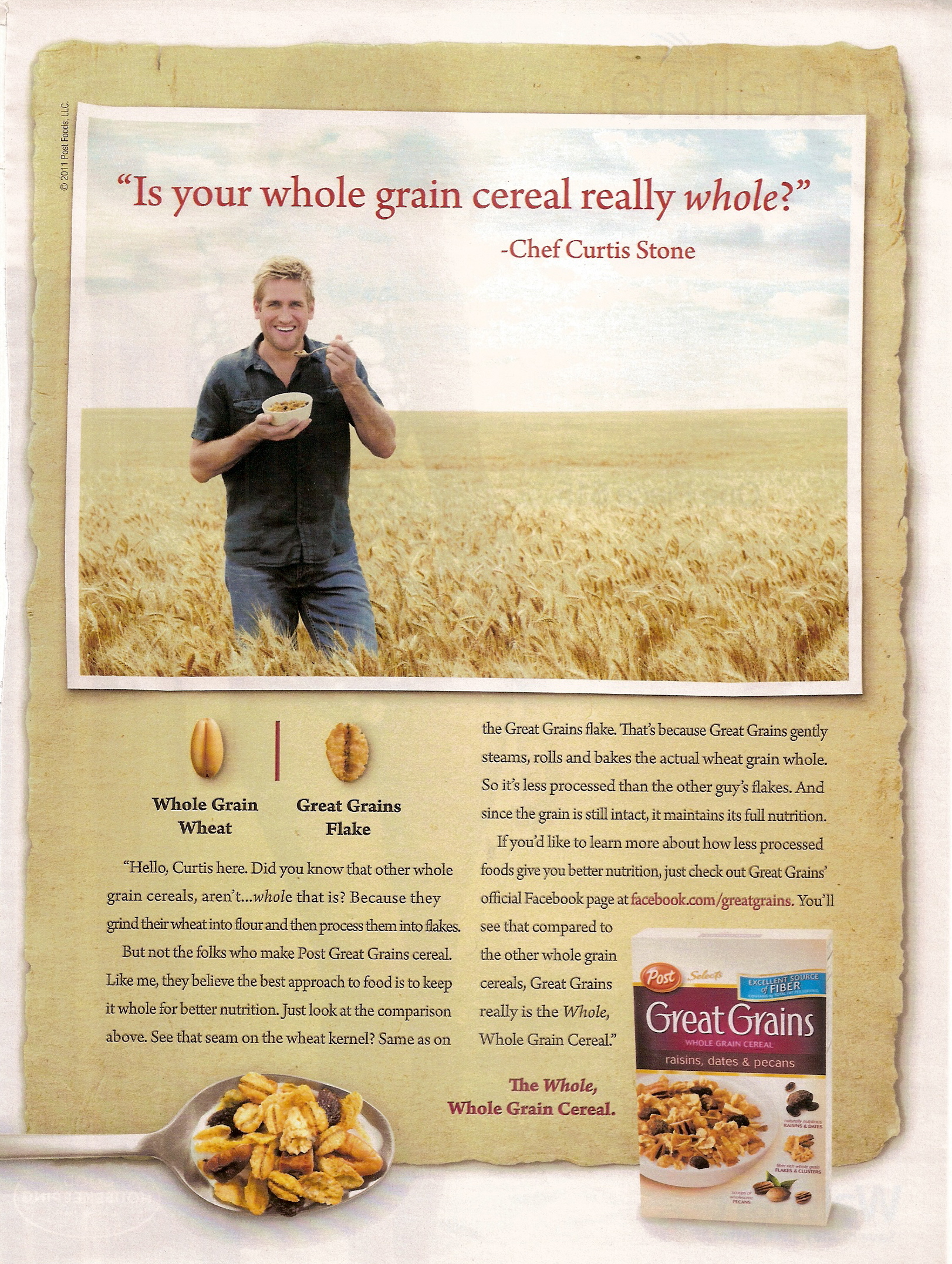The advertisement for Post Great Grains cereal features a tan background with a prominent section in the upper two-thirds showing a young man with tan golden hair, dressed in blue jeans and a dark black short-sleeve button-up shirt, standing in a wheat field. He is holding a bowl of cereal in his right hand, while his left hand is lifting a spoon toward his mouth. Above him, in bold red text, it reads, "Is your whole grain cereal really whole?" followed by Chef Curtis Stone's name. Below this, there's a further informational blurb about the cereal. In the foreground, a spoonful of the cereal, showcasing detailed oats and grains, extends horizontally from the left. To the right is an image of the Post Great Grains cereal box. The ad includes an illustration of whole grain wheat, with textual annotations pointing out "whole grain wheat" and "Grains Flake."